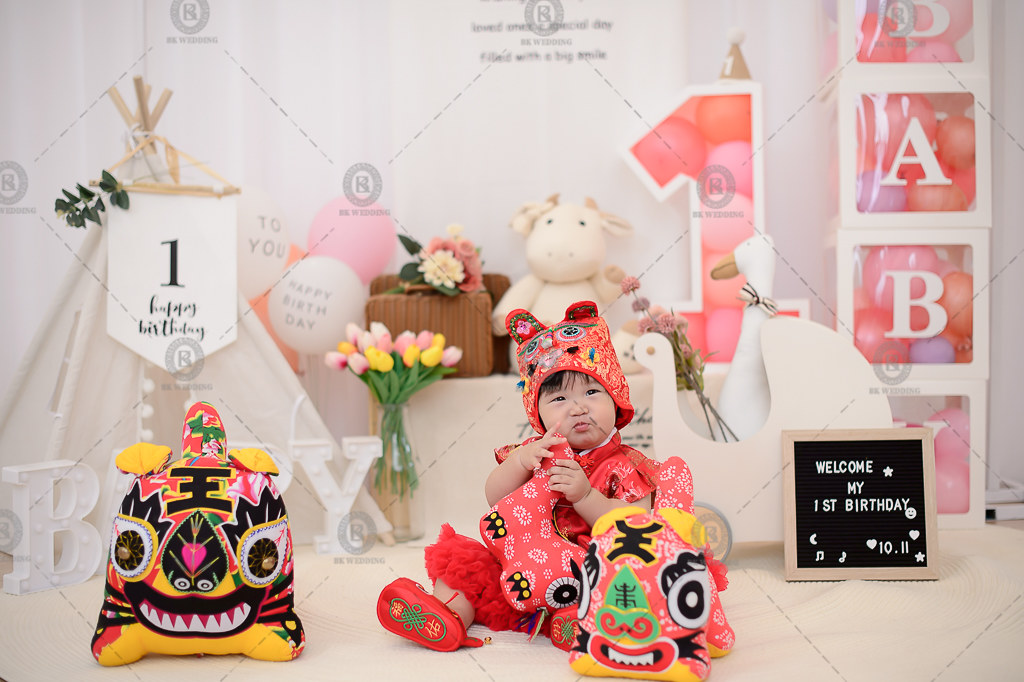In this image, we see a young child, possibly of Asian descent, dressed in traditional Chinese attire consisting of a red shirt, red flowing pants, and red shoes. The child is also wearing a distinctive pink multi-colored hat adorned with various images, featuring darker red ears. He is seated with his legs pointing towards the camera, holding a dragon-like stuffed toy in one hand.

The setting appears to be a nursery filled with various toys, including a white hippo and a stuffed piglet, with a festive birthday theme. Behind the child, there is a blackboard with a white frame and white letters that read "Welcome, My First Birthday," along with the date "10.11." Surrounding the space are decorations, such as a large, pink number one outlined in white and filled with pink balls, a banner saying "One, Happy Birthday" in cursive, and balloon-like objects resembling large white golf balls that also spell out "Happy Birthday." Additionally, to the left of the child, there is a cluster of colorful tulips in yellow, pink, and white, enhancing the celebratory atmosphere.

The toys and balloons behind the child, combined with the traditional clothing and the birthday-themed decorations, create a vibrant and joyful scene to celebrate the child's first birthday.